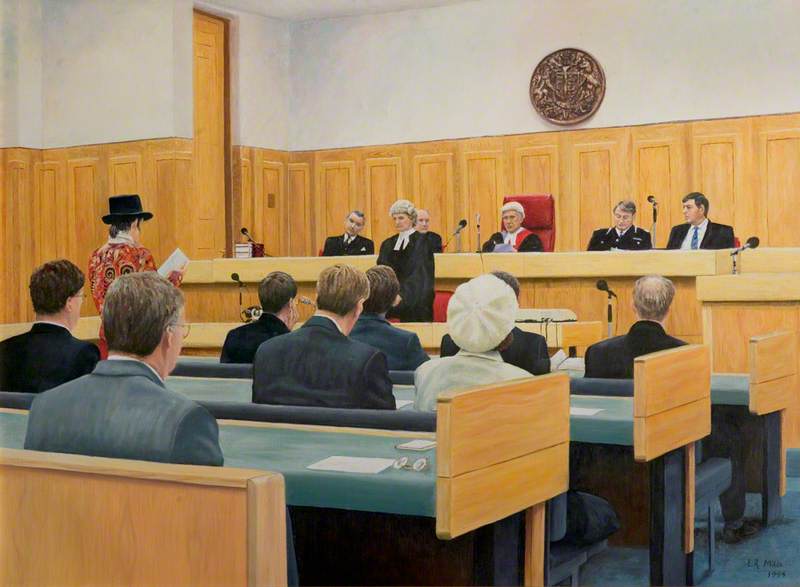The image portrays a detailed artist's rendering of a courtroom scene, potentially during a jury hearing. Dominating the scene is a judge standing in the center, donned in a traditional black robe and white scarf, her short, curly white hair adding an element of stern authority. Behind her is another seated figure, possibly another judge, positioned in a notable red chair. Flanking this seated judge are four individuals, two men on each side, all dressed in suits and sitting behind long, blue-topped tables. Microphones are positioned in front of them, hinting at their involvement in the proceedings. The background features a wooden facade with a circular golden plaque and a large wooden door to the left.

In the left foreground, a man with a white-collared shirt and a bluish-green jacket sits with his back to the viewer, obscuring his face. In front of him, three more seated figures – two men and one woman – are focused on the proceedings. The courtroom is populated with three rows of spectators or possibly jury members, all attired in formal suits, adding to the solemnity of the setting. Among them, a notable figure is a woman in an array hat and white jacket. There is also a person on the left side of the image, possibly presenting something, adding a dynamic element to the otherwise static scene. Throughout the composition, the meticulous detail captures the traditional and formal atmosphere of a courtroom, emphasizing the roles and interactions within the judicial process.